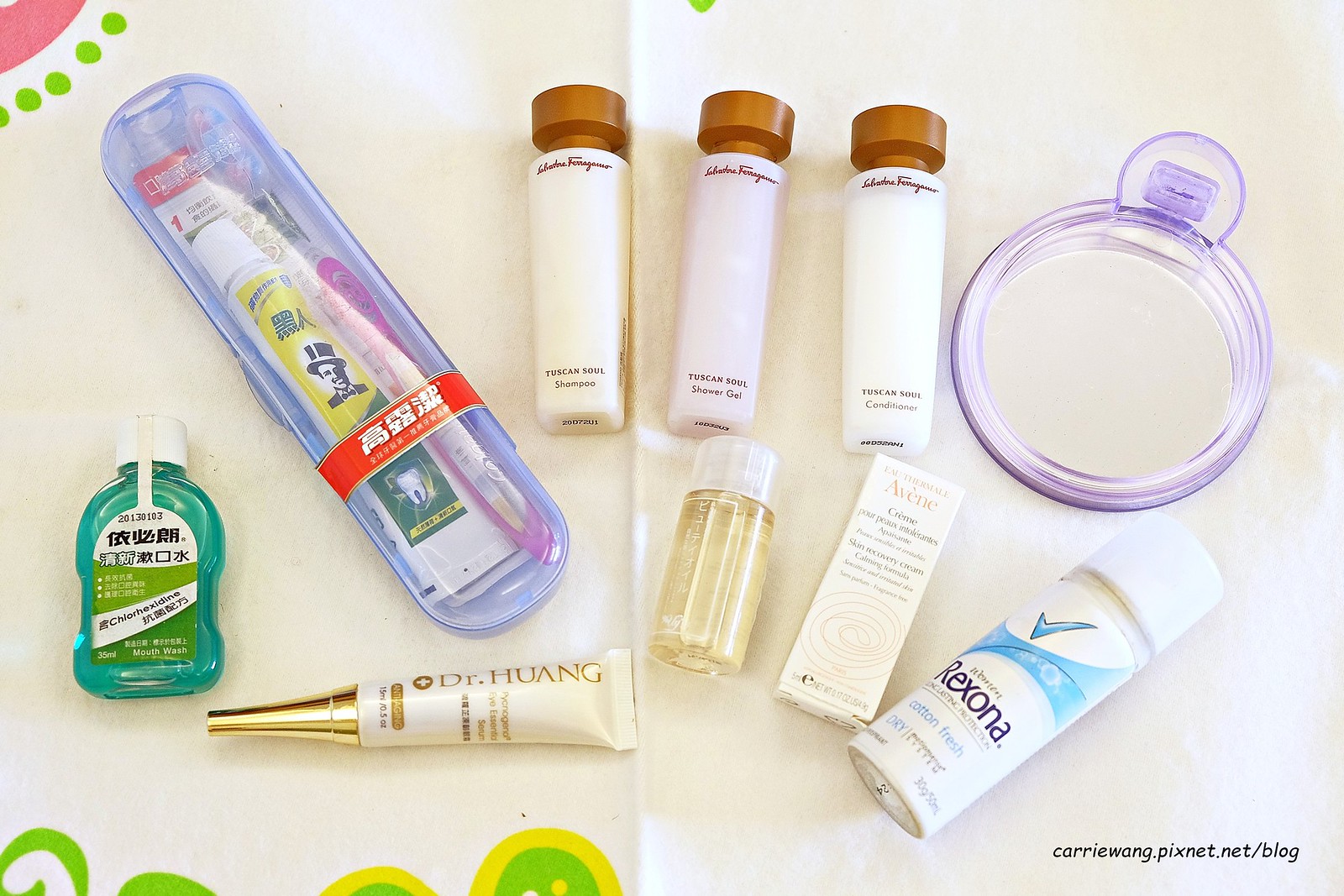The image displays an array of various skincare and personal beauty products, predominantly featuring packaging with Chinese characters, suggesting an Asian origin, likely Chinese. 

At the top left, a tiny bottle resembling mouthwash is present. To its right, a clear case contains a toothbrush and toothpaste, with a distinctive red label wrapped around it. Below this set, there is a sleek white tube with a gold tip, labeled "Dr. Huang."

The central section features three containers, each adorned with gold lids. They are labeled as shampoo (in white), shower gel (in pink), and conditioner (in white). Adjacent to these is a small clear bottle filled with an unidentified clear liquid.

Also included in the array is a compact white box, a purple plastic mirror, and a small aerosol can branded "Rexona." 

The products are placed against a white background, which appears to be tissue paper. In the bottom right corner of the image, the text "CarrieWang.pixienet.net/blog" is displayed.